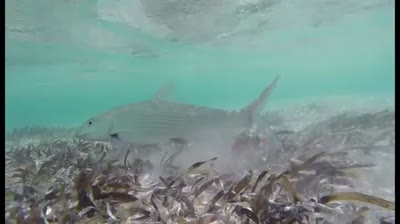This image, set underwater in the ocean, looks like a painting but could be a photograph. The scene features a single shark with black eyes, its body predominantly pale grey, swimming from right to left near the bottom of the image. Its back fin is pointed upward towards the top right corner. Surrounding the shark is a body of blue water, which transitions to a greyish hue near the opening at the top of the image, possibly due to bubbles and dirt. The water appears relatively shallow, as the surface is not too high above the shark. The foreground is filled with what looks like a lot of vegetation, depicted with grey and black brush strokes that resemble seaweed growing out of the ocean floor. The water is also described as having stirred-up particles, giving it a smoky or dusty appearance. The overall depiction emphasizes the shark as the focal point, swimming leisurely above the stirred-up ocean floor and plant life in an underwater, outdoor setting.